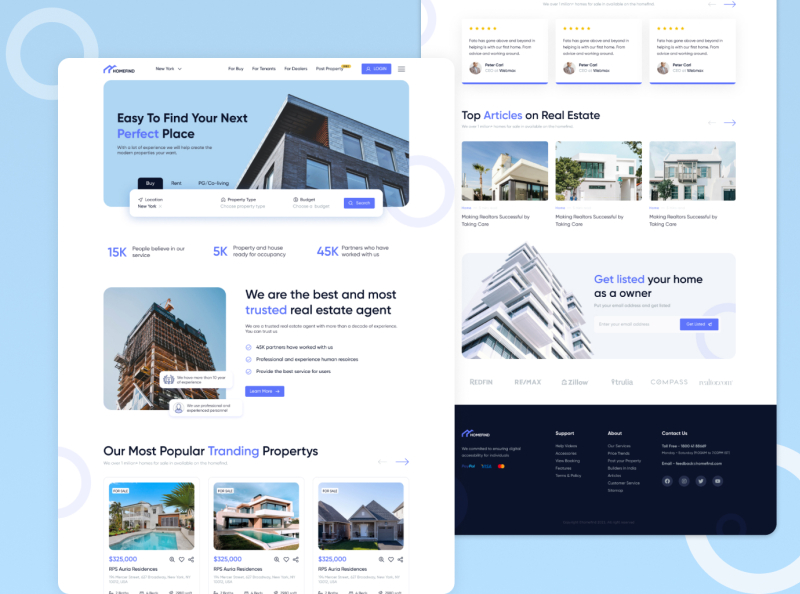**Web Page Overview - Blue Background Theme:**

The webpage features a blue background with distinct sections and elements, creating a streamlined and organized appearance. 

**Header Section:**
- Top Left: A logo resembling the letter 'M' which appears to be part of the text "Home Find" displayed prominently in bold black font. 
- Navigation: A drop-down menu titled "New Home," followed by links for "Buy," "For Tenants," "For Developers," and "Something Property."
- Login Button: Displayed in purple with white text.

**Main Banner:**
- Gray Building Image: Set against the blue background.
- Slogan: "Easy to Find Your Next Perfect Place" written in bold black text with the word "Perfect" highlighted in purple.
- Options: Buttons for "Buy Selected," "Rent," and "PG/Co-living."

**Statistics Section:**
- Metrics: 
  - "15K (15,000) People Believe in Our Service" in purple text.
  - "5K Properties and Houses Ready for Occupancy" in purple text.
  - "45K Partners Who Have Worked With Us" in purple text.

**Featured Building Image:**
- Depiction of a building under construction colored in brown, tan, and black. 
- Against a blue sky background, the phrase "We Are the Best and Most Trusted Real Estate Agent" is advertised, with "Most Trusted" appearing in purple.

**Bullet Points:**
- Points indicated with purple circles and check marks elaborating on various features and benefits.

**Property Listings:**
- Section Title: "Our Most Popular Properties" with "Properties" in bold black and "Popular" in purple.
- Images: Display of various properties, including two with pools and one with a front yard. Additional properties are shown on the right-hand side.
- Reviews: Small-sized text reviews, less legible.

**Articles Section:**
- Highlighted as "Top Articles on Real Estate" with "Top Articles" in purple and "on Real Estate" in bold black.

**Special Feature:**
- Image of a white 3D-rendered building with blue windows.
- Promotional Text: "Get Listed Your Home as an Answer" with "Get Listed" in purple and the rest in bold black.
- Search Bar: White with gray text prompting "Enter Your Email Address," accompanied by a purple button labeled "Get Started" with an arrow pointing to the right.

**Footer Section:**
- Logos: Clickable buttons for “Redfin,” “RF/Max,” “Zillow,” “Trulia,” “Compass,” and one unreadable label in gray.
- Social Media Icons: Blue circular icons for Facebook, Twitter, and YouTube set against a cyan background. 

The entire layout balances visual and textual elements to create an appealing and user-friendly experience for individuals seeking real estate services.